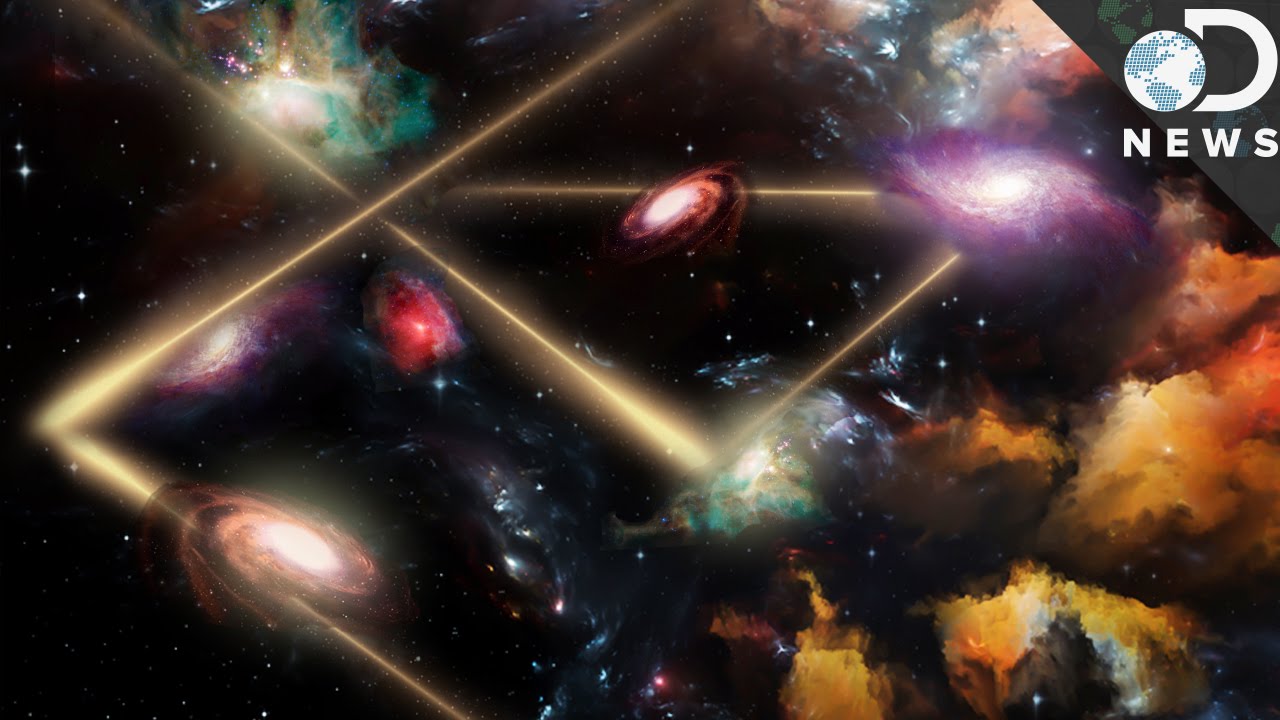The image is a detailed artistic rendition of a fantastical space scene, distinctly different from our solar system. It features several planets, each encircled by spinning, nebula-like rings accompanied by bright gaseous clouds in vivid hues of purple, orange, red, green, pink, and black. Stars are scattered throughout the scene, connected by geometric grid lines forming triangular shapes across the expanse. A logo in the top right corner reads "news" with a miniature fly depicted on one of the planets, adding to the overall surreal and imaginative feel of the artwork.